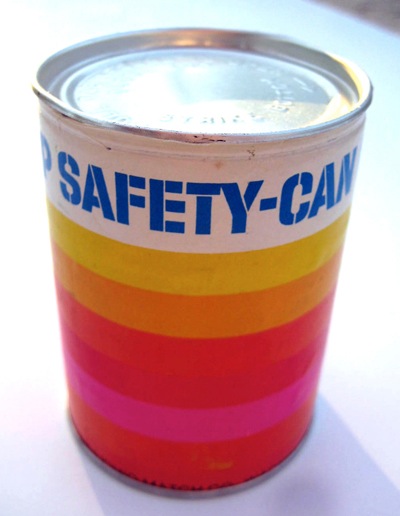This photograph captures a cylindrical tin can placed on a white surface, with its shiny, silver-colored metal lid reflecting light at the top. The can's label features bold blue stencil-type lettering that reads "SAFETY-CAN" across a wide white band situated near the top of the can. Below this band, the label transitions through several colorful horizontal stripes: yellow, orange, red, burgundy, hot pink, and another red at the bottom. Adding to the detail, there's a noticeable orange scuff mark on the lower right edge of the bottom red stripe. The lighting in the photograph comes from behind the can, casting a distinct shadow from the bottom rim that extends outward and fades towards the bottom right.